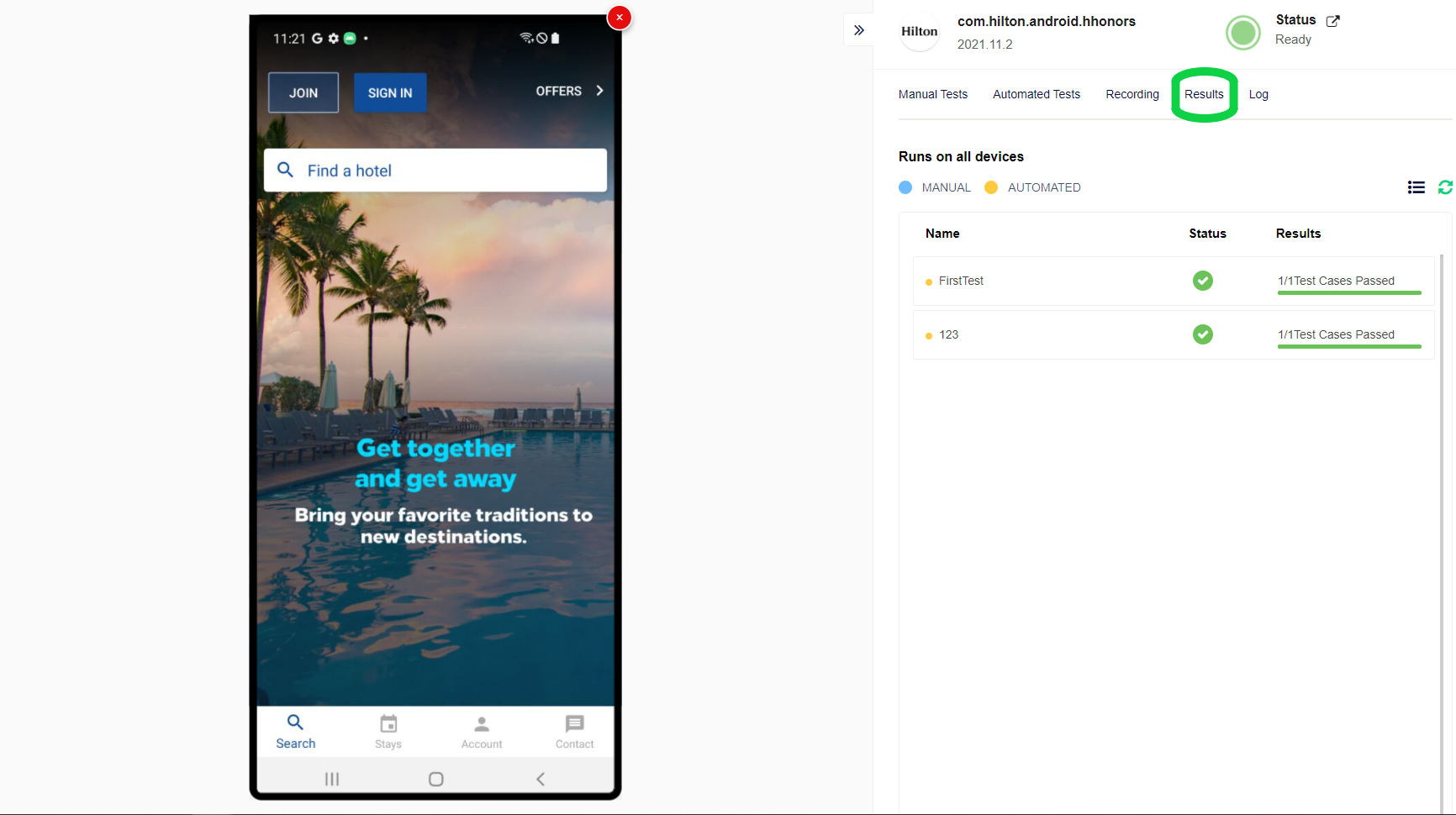This image displays a detailed view of a web page promoting a holiday destination. The scene highlights a tropical paradise featuring a large, inviting swimming pool surrounded by comfortable reclining chairs and umbrellas providing ample shade. Towering palm trees add to the tranquil ambiance, and a sky painted in pearly pink hues suggests it is evening. 

On the right side of the image, the header reads "Hilton.com" with the brand's signature double 'H' logo in front of the term "Honors." Interestingly, this header also states "Runs on all devices." Some of the headings on the web page have been clicked, although the text is very small and difficult to make out, resembling terms like "test find test 1 2 3." This indicates potential rating checks or testing elements related to the holiday destination.